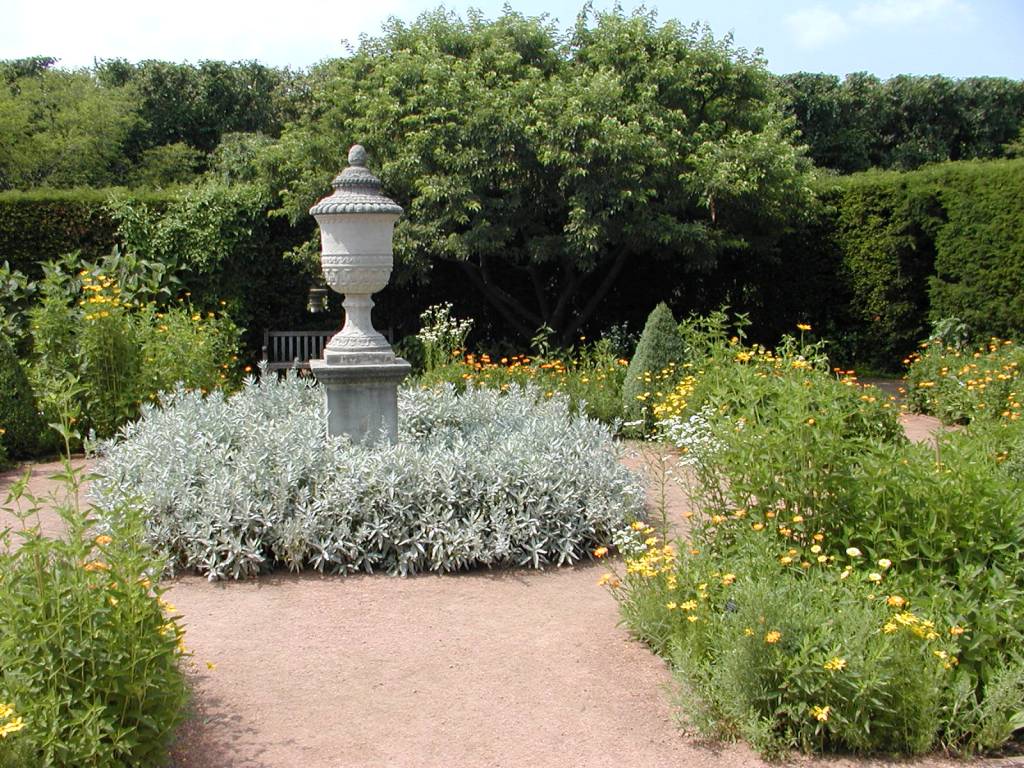This color photograph captures an idyllic garden scene bathed in sunlight. The light blue sky is dotted with various shades of white puffy clouds, from bright white to blue-gray hues. Dense greenery fills the background, comprising uniform-height trees and large, well-manicured bushes. Midway through the background, a brown tree shades a tucked-away park bench, enhancing the secluded ambiance.

The garden's focal point is a central white stone statue, resembling an urn or chalice, perched on a rectangular pedestal. This elegant sculpture emerges from a low white bush, accentuated by pale green surrounding plants. Encircling the bush and statue is a dirt path, bordered by lush green foliage adorned with clusters of yellow wildflowers.

The foreground features a mix of tall grasses and flowering weeds, contributing to the garden's natural charm. Various plants and topiaries further embellish the walkway, which guides your eye toward the prominent stone statue.

In sum, this meticulously maintained garden offers a serene and private retreat, with its carefully arranged floral displays, diverse greenery, and artistic centerpiece, all set beneath a tranquil, cloud-strewn sky.